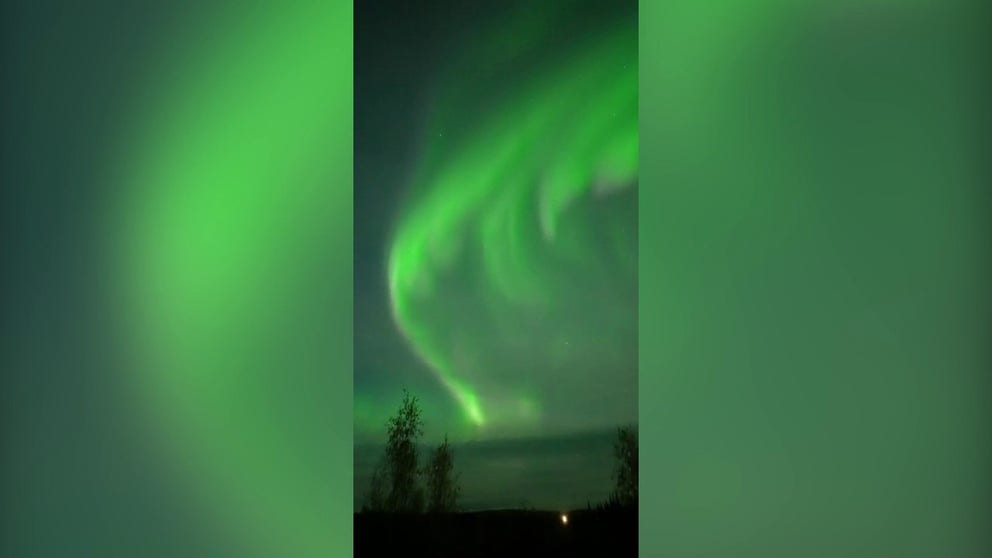This is a smartphone portrait-format photo capturing the mesmerizing Aurora Borealis, likely shot in Alaska. The photo has a vertical aspect ratio of 1080 by 1920, surrounded by a blurred, mirrored 1920 by 1080 background of the Northern Lights.

The central image, though static and vertical, is vividly clear. Dominating the sky is a stunning green aurora that curves gracefully from the bottom middle to the top right. Its neon green glow fades into a paler shade at the bottom center. The backdrop sky transitions from a deep blue near the horizon to jet black at the top. At the bottom, a darkly lit landscape with silhouetted trees frames the enchanting spectacle; two trees are noticeable on the left and a lone tree on the right, all of them casting dark, striking figures against the ambient celestial light.